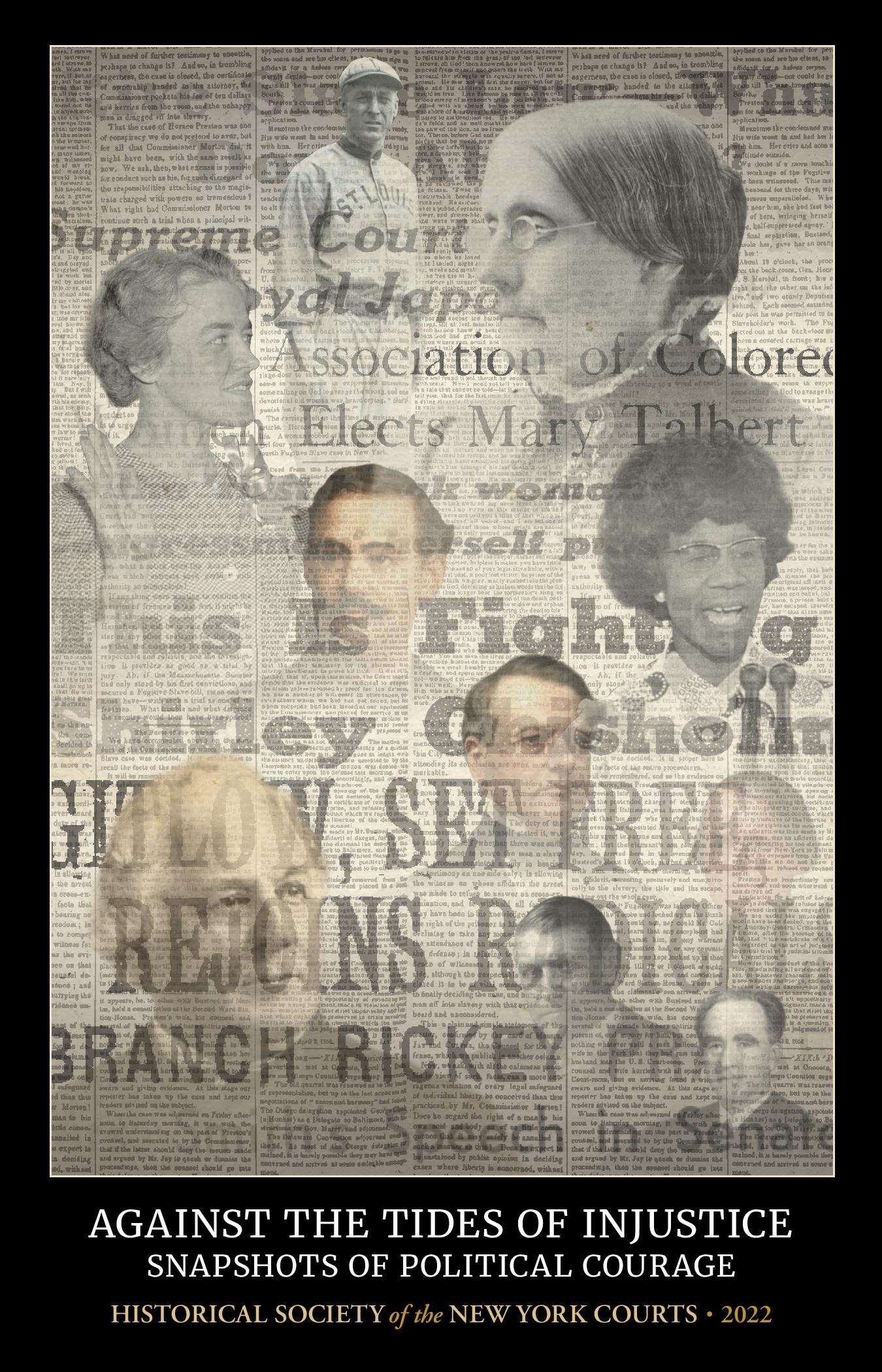The image, forming the centerpiece of what appears to be a publication, skillfully blends past and present through its design. Central to the layout are nine overlapping portraits, mixing black and white with color, which fade towards the bottom. These portraits—ranging from diverse women and men, including a baseball player, a black woman with glasses, and elderly figures—are superimposed on an evocative collage of newspaper headlines. These headlines, some partially obscured, evoke significant socio-political themes with words and phrases like "Supreme Court," "Association of Colored," "Live," "Law," "This is Fighting," "Set Free," "Rejoins," "Branch Rickey," and "Freedom of Speech." Below the image, a bold black border highlights the compelling white text: "Against the Tides of Injustice, Snapshots of Political Courage." Further down in yellow text, interrupted by the orange words "of the" in 2022, it reads "Historical Society of the New York Courts, 2022." This vivid depiction captures a multifaceted narrative of political bravery and historical resonance.